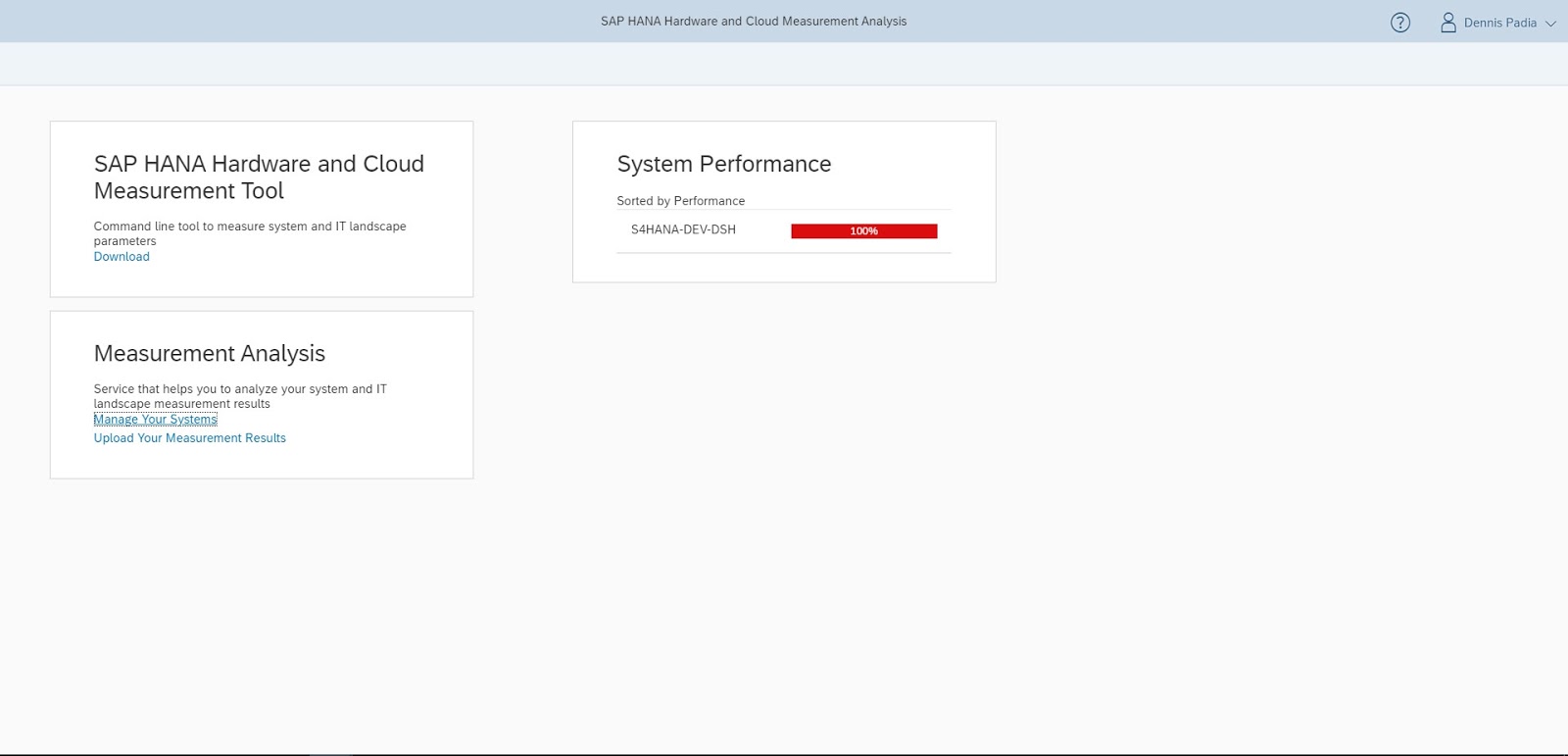In the photographic image of the web page, the layout is primarily white and blue with some black text and a prominent red button. At the top, a blue banner features the title "SAP HANA Hardware and Cloud Measurement Analysis" in black text. Within this banner, there is a circular button marked with a question mark, a profile icon to the right, and a name—possibly "Dennis P."—with a drop-down selection option.

On the left side of the page, it reads "SAP HANA Hardware and Cloud Measurement Tool" followed by a description: "Command line tool to measure landscape parameters." Below this, a blue hyperlink is provided for downloading the tool. 

In the central section, a box titled "Measurement Analysis" offers functionalities to "Manage your systems, upload your measurement results," accompanied by another blue hyperlink for further action.

Toward the lower part of the page, there's a box labeled "System Performance" which is sorted by performance type. Within this section, "SAP HANA Dev OSH" is noted, along with a hard-to-read red button.

Overall, the web page appears to be structured to provide tools and resources for SAP HANA's hardware and cloud performance measurement.